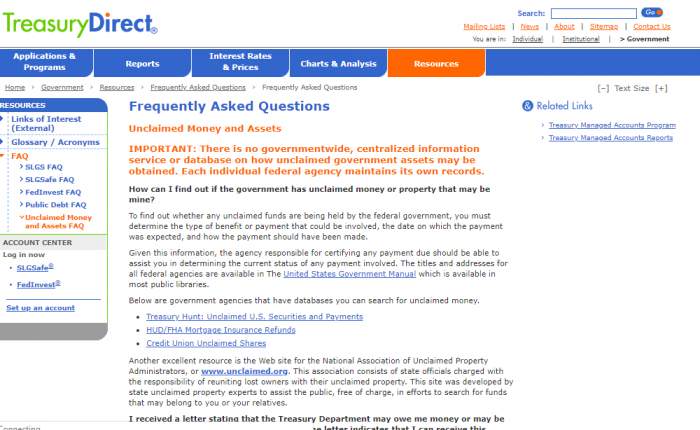Screenshot of a Government Treasury Website

The image is a screenshot of a government treasury website featuring a minimalist design. The background is primarily white. In the upper left corner, the website's logo prominently displays "Treasury" in orange font followed by "Direct" in blue font. Positioned in the upper right corner, a small search field and a sitemap can be seen, offering easy navigation options such as links to the mailing list, news updates, the sitemap, and contact information. Users can select if they are individuals, institutions, or governmental entities.

Directly below this, a row of blue rectangular buttons with white font is present, labeled as follows: "Applications and Programs," "Reports," "Interest Rates and Prices," "Charts and Analysis," and "Resources." The "Resources" button is highlighted in orange, indicating it is currently selected. Below this navigation bar is a broad white page.

On the left side of the page, there is a navigation menu under the "Resources" category. This menu includes options such as "Links of Interest," "External," "Glossary and Acronyms," "FAQ," and various sub-categories of FAQs related to SLGS and Fed Investment, Public Debt, and Unclaimed Money and Assets. Additionally, there are options to access the "Account Center," "Wagon Now," "SLGS SAFE," and "Fed Invest" sections, with an option to "Set up an Account."

To the right of this menu, the content area lists "Frequently Asked Questions" specifically about "Unclaimed Money and Assets." 

This organized and user-friendly layout allows for easy navigation and access to various treasury-related resources and information.